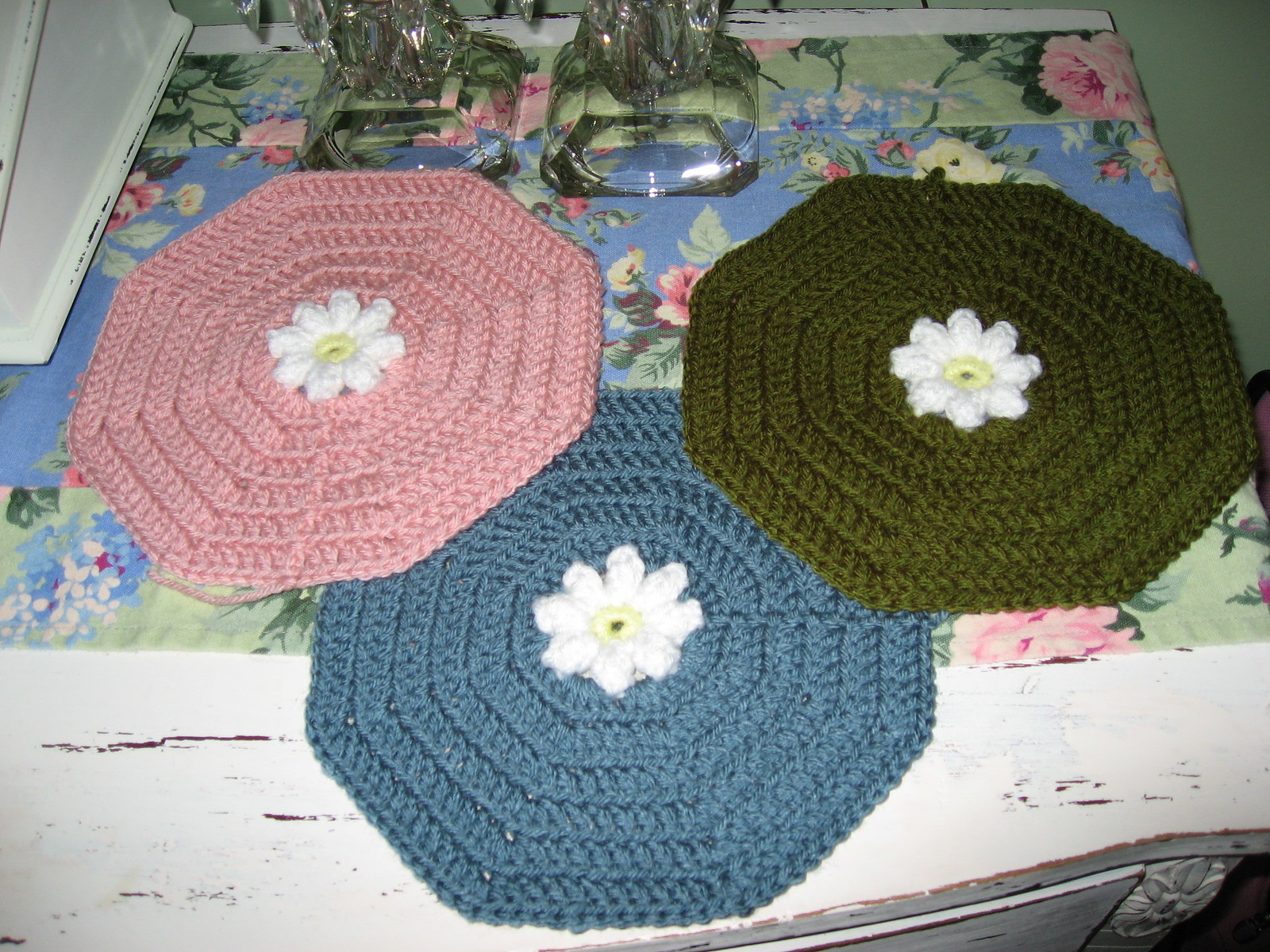The photograph depicts a collection of handcrafted, crocheted placemats, intricately designed with white flowers at their centers, each featuring a small green spot as the core of the flower. There are three placemats: one pink, one blue, and one deep green, all octagonal in shape and woven in a circular pattern. These colorful placemats are arranged on a slightly worn white table, covered with a matching tablecloth that also displays a floral motif in the same pink, blue, green, and white colors. The tablecloth, resting across a dresser or countertop, is accompanied by clear images believed to be candlesticks, adding to the cozy, vintage ambiance of the setting.